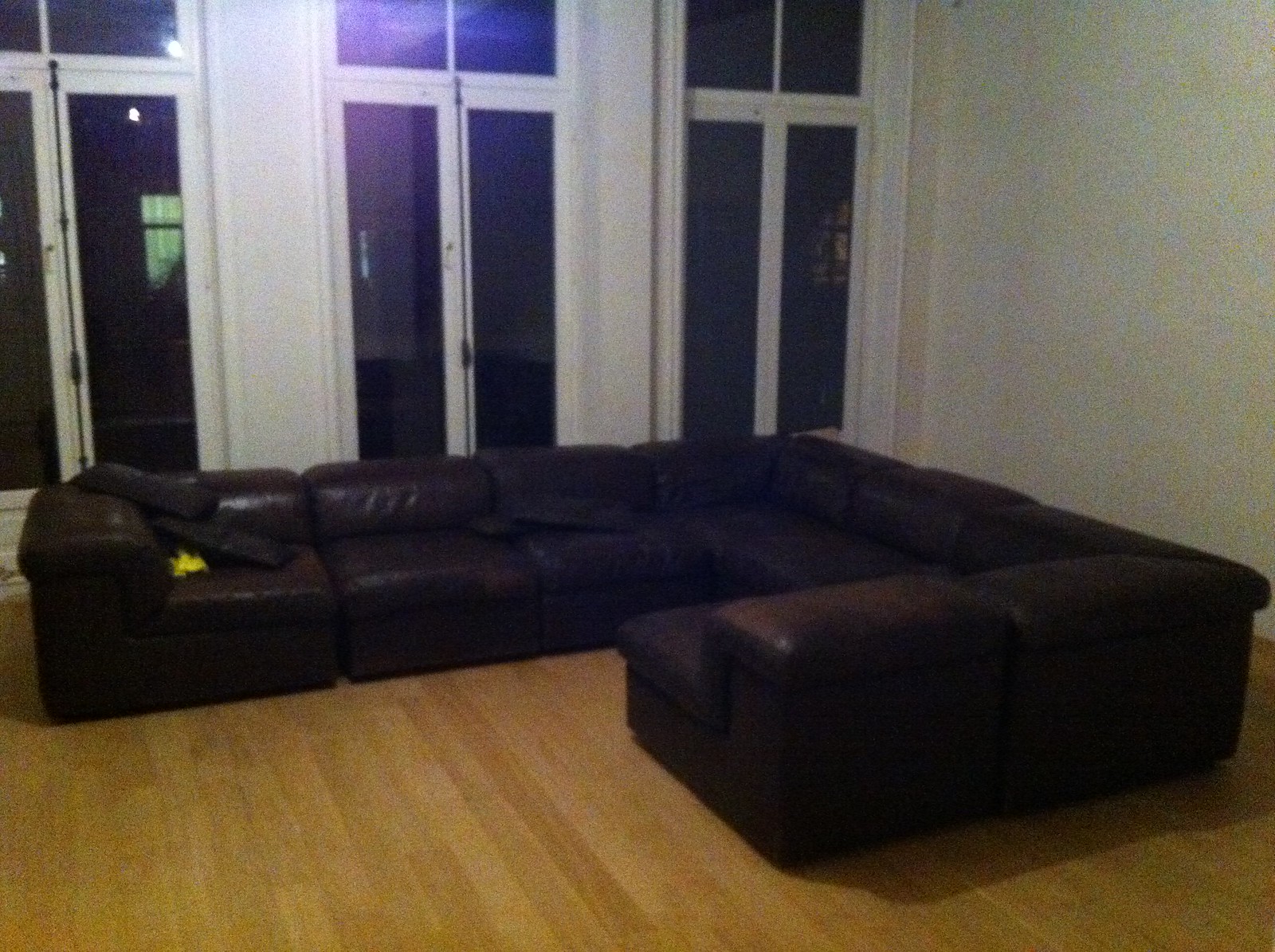The image depicts a living room with a worn and aged dark brown leather sectional sofa, prominently positioning as the room's focal point. The sofa, featuring scuff marks and visible damage, including exposed stuffing on the far left seat, forms an L-shape, almost U-shaped but with walking space around it. The back is slightly low, and the seating includes cushions with a yellow, fluffy item at one end. The room's flooring consists of light blonde brown wooden boards, complementing the white walls. Behind the sofa, there are three sets of French doors, each flanked by windows, framed in white, and separated by wall sections and a noticeable black wooden pole in the middle set. It is nighttime outside, and through the doors, another house with a lit window and green curtains is visible. The room is otherwise sparse, accentuating the large, rather decrepit sofa as the primary feature.